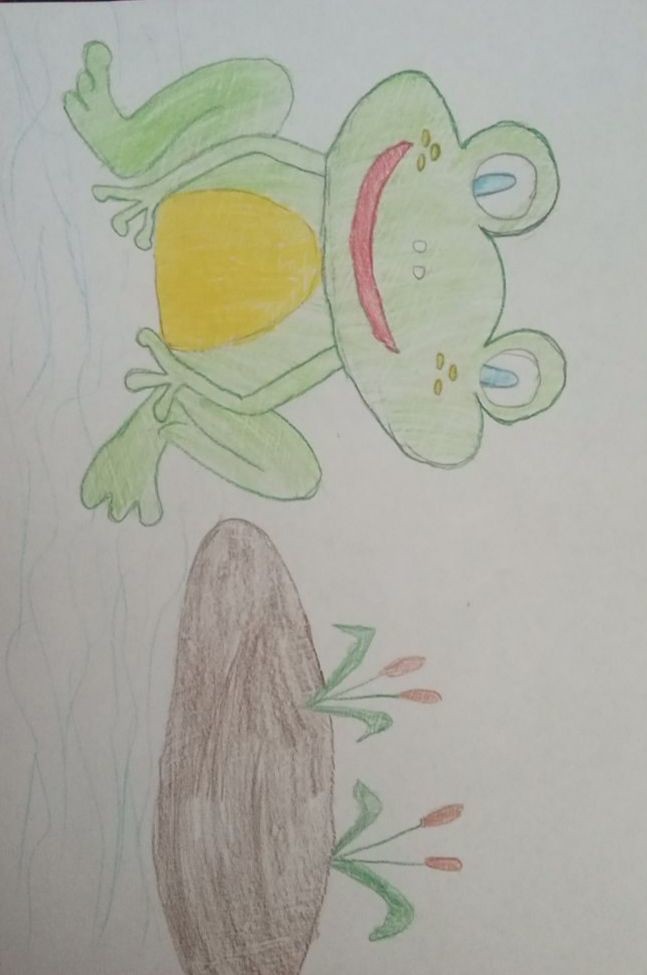This charming child's drawing features a cheerful green frog with a yellow belly and a broad, red crescent-shaped smile, positioned at the top of the picture when viewed from the side angle. The frog's face is adorned with white circular eyes, each containing a blue oval, and it's surrounded by three green dimples or freckles on each side of its mouth. The frog sits on wavy blue lines, suggesting it’s afloat on water. To its left, there is a brown mound or lily pad, complete with green stems and vibrant red flowers, likely tulips. The frog's playful and happy posture, coupled with its cute legs and arms, adds to the whimsical and endearing nature of the drawing.